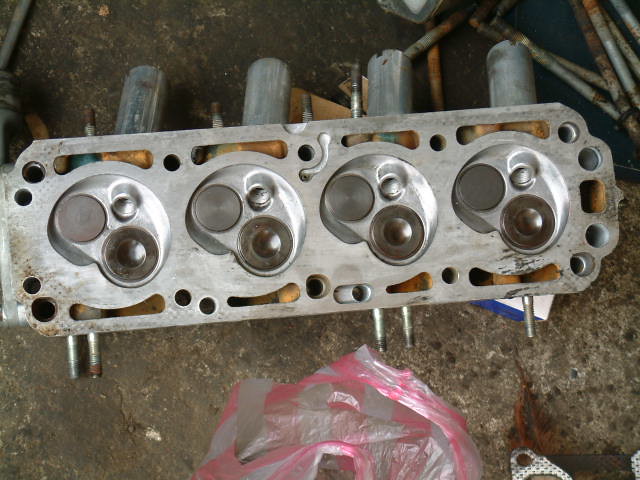In this digital photo taken in what appears to be an indoor setting, a mechanical device, likely a head from an engine, is prominently displayed on a dirty, gray concrete floor. The concrete, marked by the aggregate stones within it, seems older and damp, especially towards the top portion of the image, reflecting a darker and grimier appearance. The metallic device in the center has a distinctive silver color and features four prominent half-circle sections in the middle. Each half-circle has a solid metal piece on the upper left side and a duller metal piece with a divot on the lower right side. Surrounding the edges, the device is straight on the sides and two-layered on the ends, punctuated with multiple holes and eight elongated hole punch-outs. Four pipes extend from the top edge, while a couple of inlets are visible along the bottom edge. The mechanical apparatus rests amid scattered pipes and other materials on the ground, including a white and pink-striped plastic bag at the bottom. Metal rods, extremely dirty and gray, are situated in the upper right portion of the photo, while additional rusted metallic tubes and some wooden elements are visible in various parts of the image.